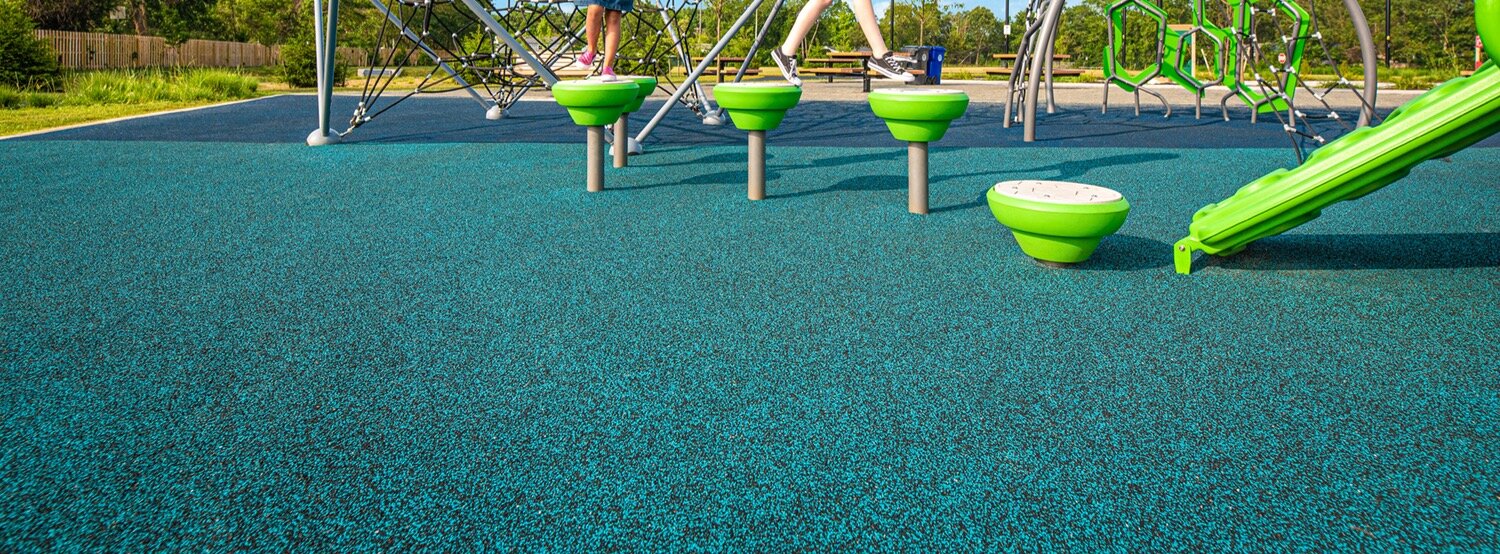The photograph captures a vibrant playground scene during the day, emphasizing the colorful and engaging environment designed for children's play. The foreground is dominated by a lush, green artificial grass surface with a prominent green slide to the right. This slide descends towards the center of the image. Spaced around the slide are four distinct, green-topped fixtures resembling upside-down plungers, elevated on brown poles at varying heights, functioning as landing pads or stepping stones.

In the midground, the feet of two children are visible; one wears black sneakers, the other appears in either pink Vans or possibly barefoot, emphasizing the playful activity occurring in the space. The background features a substantial metal and silver-colored jungle gym where additional kids are climbing, their feet in black sneakers clearly noticeable, while the rest of their bodies are cropped out. Also visible are elements suggesting various playground equipment, potentially including trampolines and step boards, contributing to the lively atmosphere.

The scene is framed by small patches of grass and bushes, with picnic tables on concrete and a brown wooden fence visible to the left. Trees in the background provide a natural backdrop, rounding off this detailed snapshot of a bustling, colorful playground.